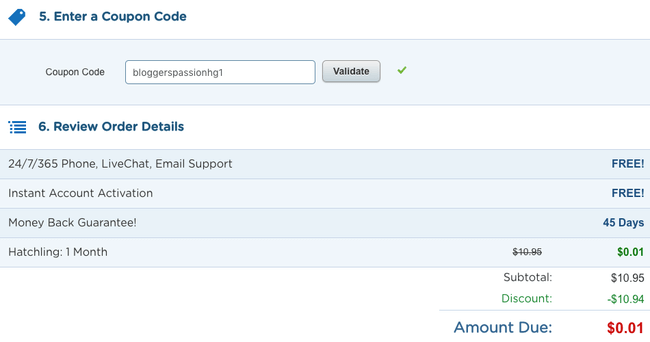The image showcases the final stage of an online checkout process. The user has entered the coupon code "BLOGGERSPASSIONHG1" into the designated field and clicked the "Validate" button, which resulted in a green check mark indicating the successful application of the discount. The order details are displayed below, listing various line items and their respective costs. Initially, the "Hatchling - One Month" service was priced at $10.95, but the coupon code has reduced the cost to just one cent. Additionally, the image highlights features of the service such as a 45-day money-back guarantee, 24/7 customer support via phone, live chat, and email, as well as instant account activation. The "Hatchling" service appears to be an online offering, likely related to web hosting or a similar internet-based service. The total amount due is clearly shown to be $0.01.